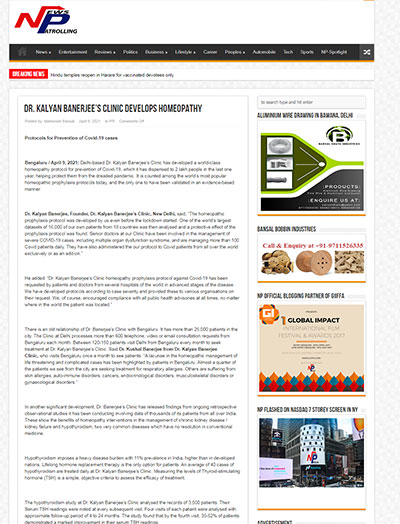This screenshot captures a web page from the "News Patrolling" website. At the top of the page, "News Patrolling" is prominently displayed. Beneath this, there is a black banner with white text that is too blurry to decipher. The headline below the banner reads, "Dr. Kalyan Banerjee's Clinic Develops Homeopathy." An article is present under the headline, but the text is too small and blurry to be legible, even when enlarged.

To the right side of the screenshot are several photographs accompanied by descriptions, all of which are too blurry to read. The first photograph displays three small black-and-white images set against a green background. The second photograph appears to feature wooden spools or similar objects. Below this is a text-only image, illegible due to its small size. The bottom photograph shows a large city street, devoid of visible people or animals. The writing on this photo is also too small to read, even when enlarged on the monitor.